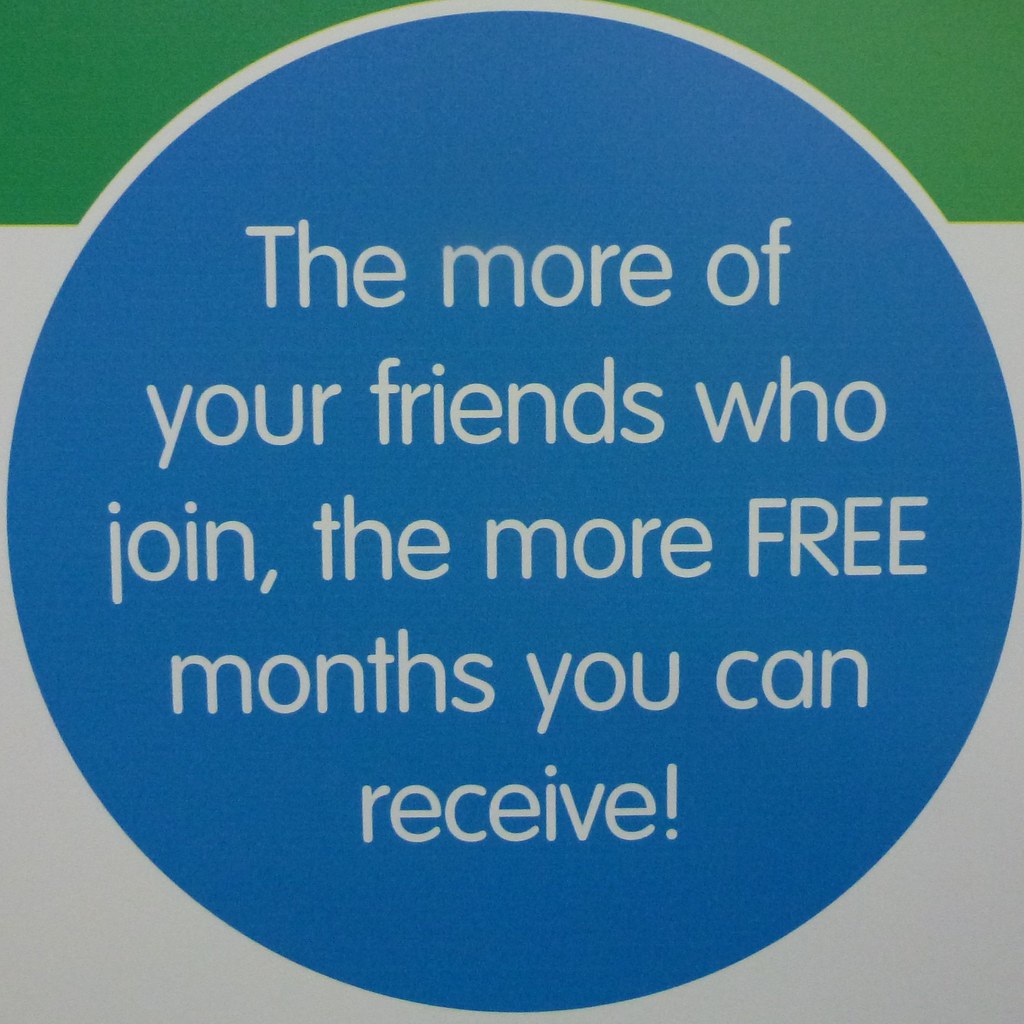The image features a promotional banner or poster with a two-toned background, divided into a top fourth that is green and the remaining three-fourths that are white. Dominating the center of the image is a large blue circle. Inside this circle, in white text, the message reads: "The more of your friends who join, the more FREE months you can receive!" with "FREE" notably capitalized. The banner appears somewhat poorly printed, exhibiting some noise and imperfections.